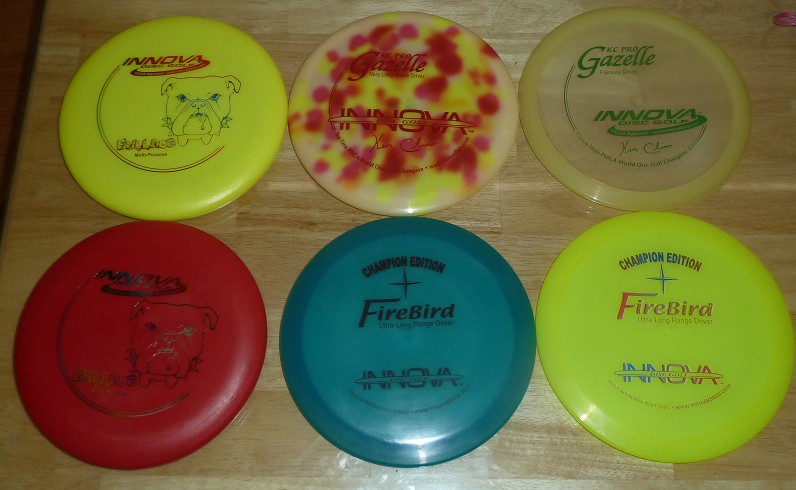The photograph features a collection of six distinct frisbees laid out on a wood-textured surface, characterized by its uneven tones and beach-like coloration. The frisbees are arranged in two imperfectly aligned rows of three each. 

In the top row:
1. The leftmost frisbee is a bright yellow one, adorned with a blue bulldog and red "INNOVA" text.
2. The middle frisbee is yellow with heavy red splotches and the text "INNOVA" in red.
3. The rightmost frisbee is a pale, translucent yellow, allowing the table to show through, and it reads “GAZELLE” and “INNOVA” in yellow letters.

In the bottom row:
1. The leftmost frisbee is red and features a silver bulldog along with the text "INNOVA."
2. The middle frisbee is turquoise and marked with "FIREBIRD" and "INNOVA" in black text.
3. The rightmost frisbee is a vibrant neon yellow, prominently displaying “CHAMPION EDITION FIREBIRD” and "INNOVA" in blue and red text.

Overall, the unique colors and intricate designs of these frisbees contrast beautifully against the warm, earthy tones of the wooden surface.